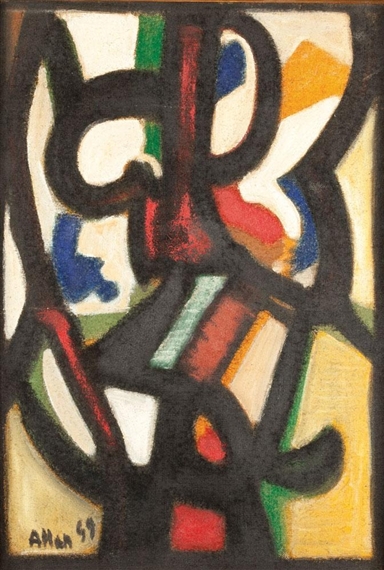The abstract painting predominantly features a series of broad black graffiti-like lines winding over a white background, creating a dynamic composition across the canvas. Additional colors include scattered blue, red, yellow, and green elements, with deep blue figures on both the left and right side, one resembling a crouching person. The top right corner contains a striking yellow triangle, while a green line marks the top left. The image's bottom half is accentuated with a red line, interspersed with green and yellow stripes, and tan corners on the lower right and left. Amidst the colorful swirls and blob-like shapes, which some might interpret as facial features, the lower left corner bears a signature reading "Aham 59," suggesting the artist's name and the year of creation. Overall, the painting exudes an impressionist style with a chaotic yet harmonious blend of colors and forms.